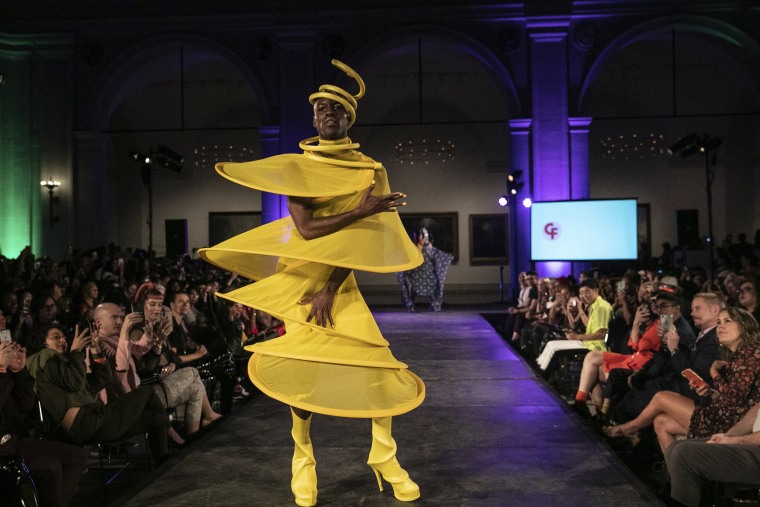This full-color photograph, taken indoors, vividly captures a controversial fashion show set against a brown wall decorated with framed pictures. The square image features a runway running vertically through the center, flanked by large groups of spectators on both sides, many of whom are busy taking photographs. The scene is illuminated with striking purple lighting, both on the floor and from multiple archways in the background. Notably, on the right-hand side, a TV screen with a blue background is visible.

Commanding the viewer's attention is an African American model located front and center. The model is dressed in an extraordinary yellow ensemble composed of hoops connected by see-through fabric that spirals upwards from the knees to form a twisting headpiece. Adding to the audacious look are knee-high, high-heeled yellow boots, detailed with six-inch heels. Behind this model, another figure in similarly avant-garde attire can be seen, adding to the surreal atmosphere of the event. The setting appears to be an auditorium, complete with pillars and a distinctive runway, all illuminated by a palette of green and purple lights.